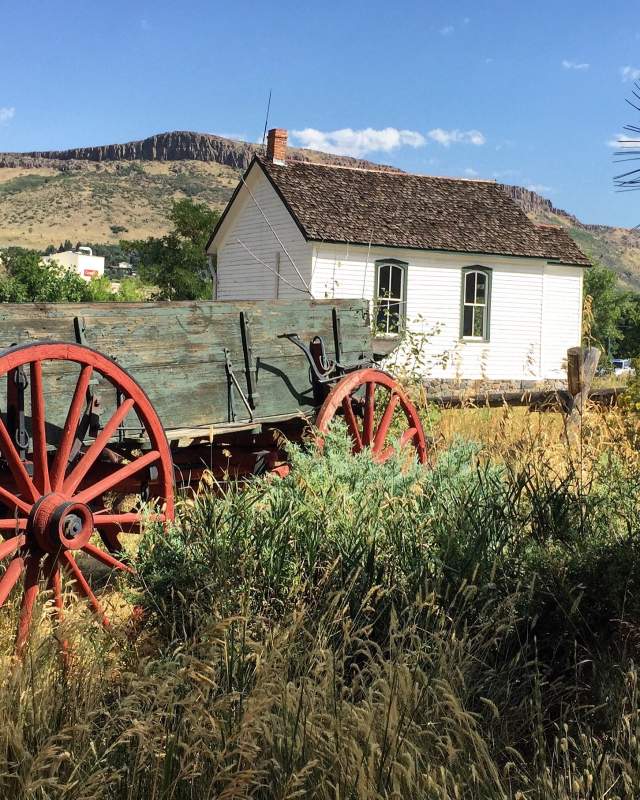In a picturesque rural setting, a rustic wooden wagon dominates the foreground, featuring two large, strikingly red wheels and a weathered, greenish wooden bed of unknown purpose. Behind the wagon stands a diminutive, one-story building characterized by its white wooden siding, a quaint clay-tiled roof, and a sturdy brick chimney. The backdrop reveals a majestic mesa or plateau, with steep cliffs rising dramatically against the clear, sunny sky, dotted with only a few scattered clouds. This scene captures a moment of serene simplicity and timeless beauty.